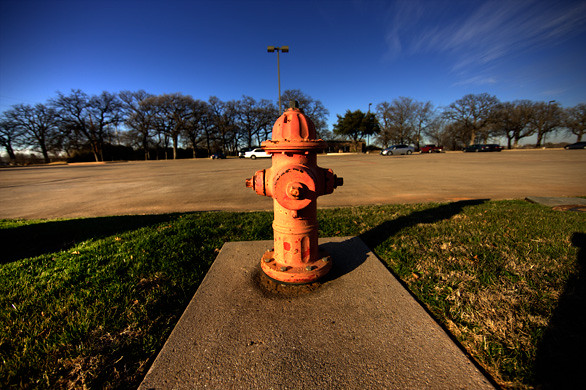In this rectangular outdoor daytime photograph, the focus is a slightly rusted, aged red fire hydrant with patches of yellow, situated on a small gray concrete slab nestled in a patch of short, somewhat grayish, trimmed grass. A large parking area or road lies in front of us, shadowed to the rear right by the fire hydrant, indicating the sun is positioned behind and to the left. The mid-ground is characterized by several cars parked near a gently curving line of trees that extends along the horizon. The backdrop consists of a clear, deep blue sky with faint air streaks and a towering floodlight, reminiscent of those found in sports fields, standing tall among the trees.